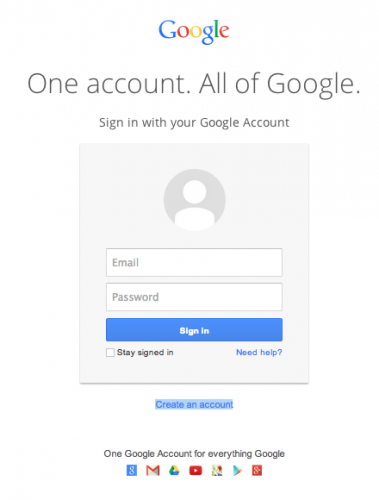The image features a centered layout on a completely white background. At the top is the iconic Google logo, showcasing the typical pattern of colors: blue, red, yellow, blue, green, and red, spelling out "Google". Below the logo, in large black font, the text reads: "One account, all of Google." 

Further down, in a font that is approximately one-quarter of the size of the previous text, it says: "Sign in with your Google account." Beneath this text, there is a grey rectangular sign-in form. The form includes an empty profile picture placeholder, and fields for entering an email address and password. A blue button with the text "Sign in" written in white is featured prominently within the form.

To the left of the sign-in button, there is a checkbox labeled "Stay signed in." On the lower right of the form, a blue text link with the word "Help?" is displayed.

Below the sign-in form, highlighted in light blue, is a call-to-action link that states "Create account" in dark blue text. At the very bottom of the image, in black text, it says: "One Google account for everything Google." This is accompanied by various icons representing different Google apps.